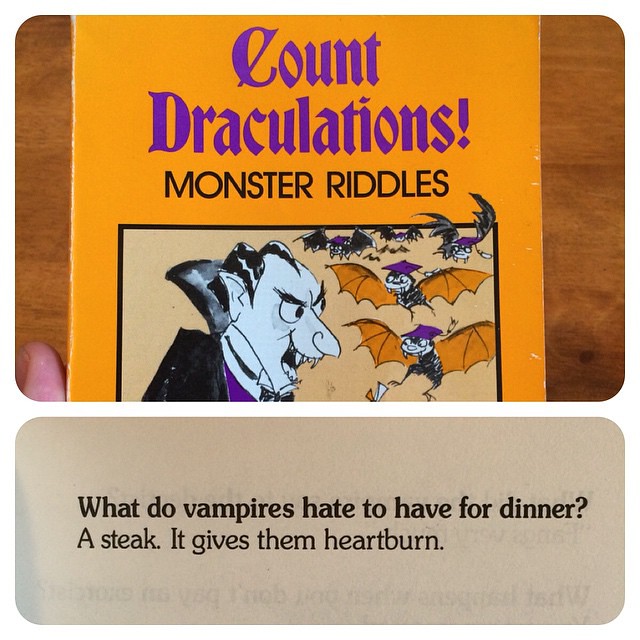The image depicts a vintage monster riddle book, likely from the 70s or 80s, with a soft yellow cover. At the top, the title "Count Draculations!" is prominently displayed in a striking purple, Gothic-style font. Beneath it, in a more modern black font, reads "Monster Riddles." The cover features a whimsical hand-drawn illustration of a classic Dracula-like character, complete with a wide cape and distinctive neck extension, gazing at a mix of bats. Some of these bats are humorously adorned with purple graduation caps, have orange wings, black bodies, and fangs, suggesting they might be tiny vampire bats. A few smaller, crudely drawn black bats also flit above them. The book cover image is framed by a small black border, and a white thumb is visible, indicating someone is holding the book against a light yellow wooden desk. Below this, there's another rounded-corner box with a gray background containing a sample riddle from the book: "What do vampires hate to have for dinner?" followed by the punchline, "A steak. It gives them heartburn."